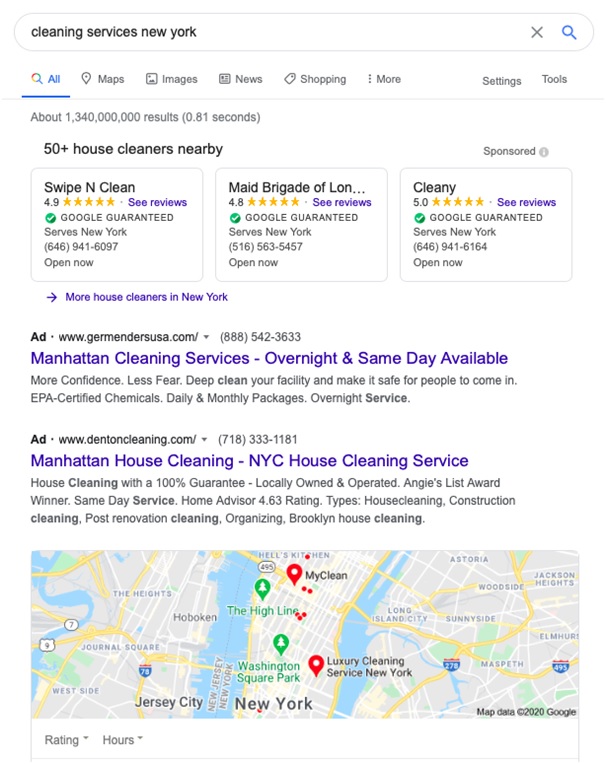This image captures a screenshot from a Google search results page where the user has typed in "cleaning services New York". Displayed under the "All" tab, the search results highlight over 50 local house cleaning services. At the top, three prominent cleaning services are showcased in rectangular boxes. 

1. **Swipe and Clean** has an impressive rating of 4.9 stars and provides services within New York.
2. **Maid Brigade of Lu**, (the full name is not displayed and ends with an ellipsis), boasts a 4.8-star rating and also serves the New York area.
3. **Kleene** stands out with a perfect 5.0-star rating. This entry indicates that the business is Google guaranteed, includes contact details, and notes that it is currently open for service.

Below these listings, there is an option to view additional house cleaners in New York. Two advertisements are positioned at the top of the search results:
- One for **germanderusa.com**, offering services in Manhattan.
- Another for **dentoncleaning.com**, also catering to Manhattan Cleaning Services.

The bottom of the image features a map of New York, giving a visual reference to the service area for the listed cleaning companies.